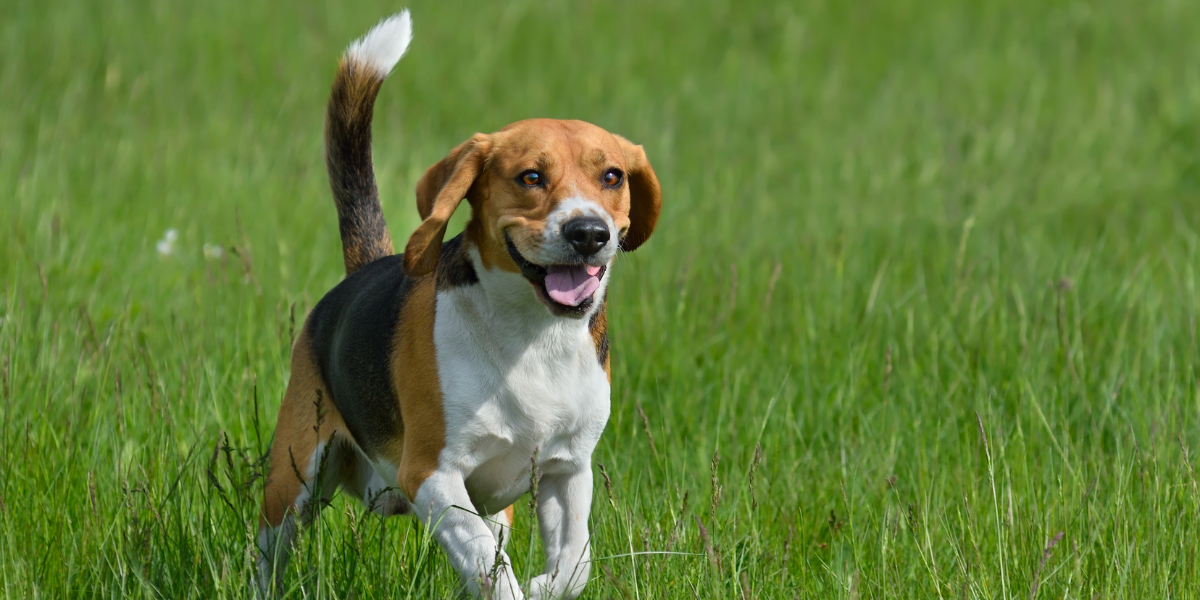The image captures a vibrant outdoor scene, dominated by a lush expanse of green grass, interspersed with occasional brown strands and white dots in the blurred background. A small dog, full of energy and joy, is depicted running from the left towards the right, slightly to the left of the image’s center. The dog’s brown face, adorned with expressive brown eyes and an open mouth showcasing a pink tongue, radiates excitement. Its ears are floppy and brown, and its front paws, belly, and the lower part of its back legs are white. The dog's back features a mix of brown and black, with its tail raised high, displaying a black and brown coloration with a distinctive white tip. Sunlight illuminates parts of the dog, further highlighting its vibrant, varied coat against the rich green grass of the sunny field.